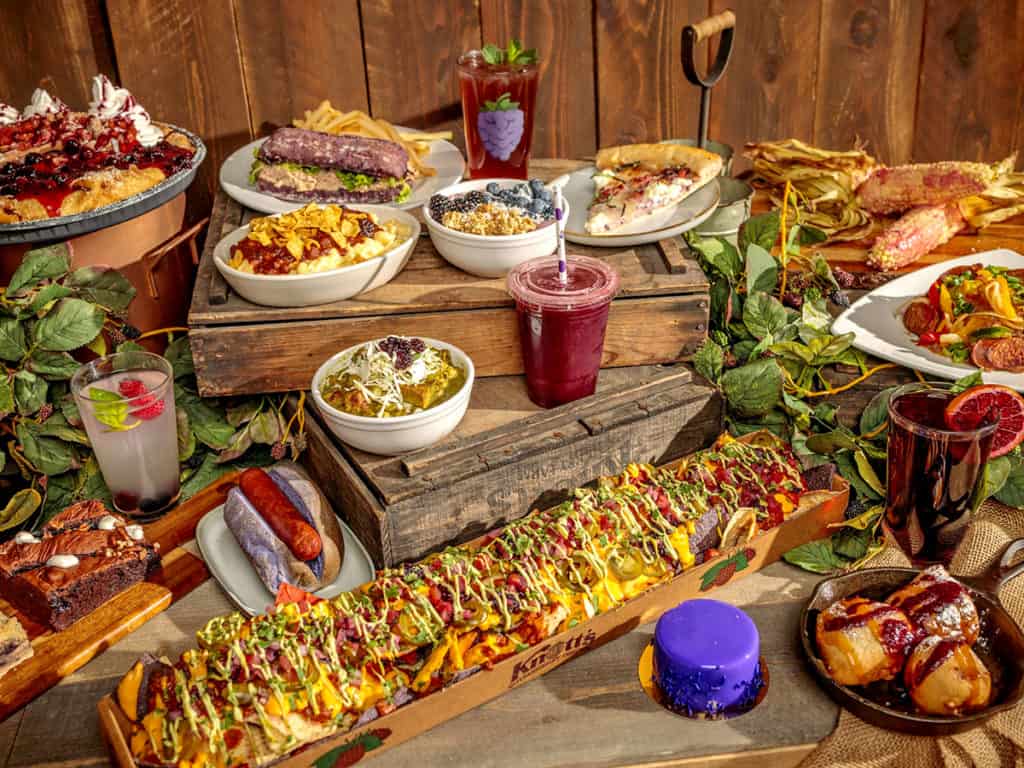The image depicts an abundant and colorful feast set up on a wooden table, positioned against a wooden wall or fence. The table is loaded with an array of appetizing foods, combining elements of Mexican cuisine with various other dishes. Notably, there is a large tray filled with nachos or nacho fries, an assortment of tacos, bowls of green chili, and what seems to be a long sandwich or a row of hot dogs. Additional items include a slice of pizza, fried dough, sandwiches, waffles, and a sizable chocolate brownie. Drinks are also plentiful, including a purple smoothie in a clear plastic cup, a white beverage with berries, and a big glass of iced tea. Garnished with green leaves and corn husks for either decoration or consumption, the setup is bright and inviting, arranged meticulously on the wooden table. The scene is rich in detail, with wooden boxes and vines accentuating the lush, vibrant spread of food.